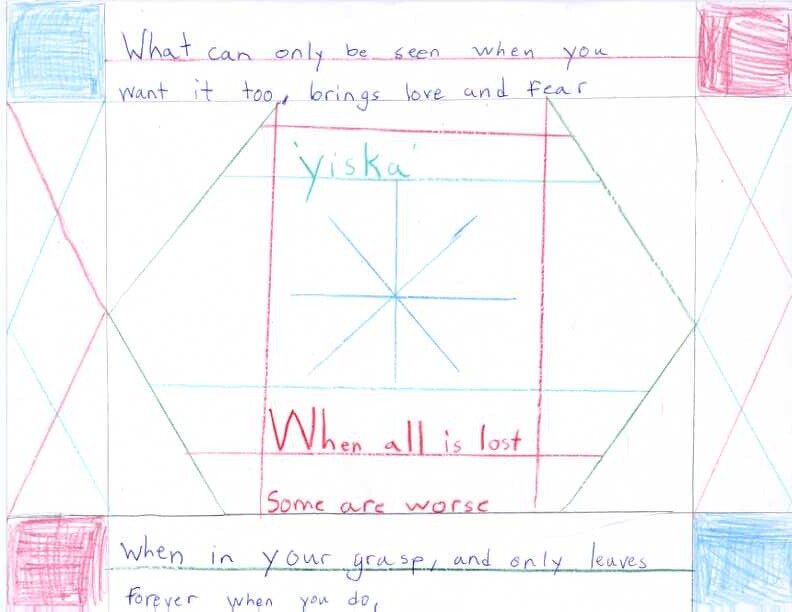The image is a hand-drawn diagram on white paper, featuring distinct colored elements and text in each corner and within the center. In the top left and bottom right corners are blue squares, while the top right and bottom left corners feature red squares. Between the blue and red squares in the top half of the image, there are two lines of text reading, "What can only be seen when you want it to brings love and fear." Below this text, centered at the top, is the word "Jiska" in blue font. Beneath "Jiska," in red font, is the phrase, "When all is lost some are worse." In the lower half of the image, two lines of text are positioned between the red and blue squares, stating, "When in your grasp and only leaves forever when you do." Red and blue lines crisscross towards the center of the image, converging at a blue star. The combination of colored squares, crisscrossing lines, and evocative text creates a visually striking and meaningful composition.